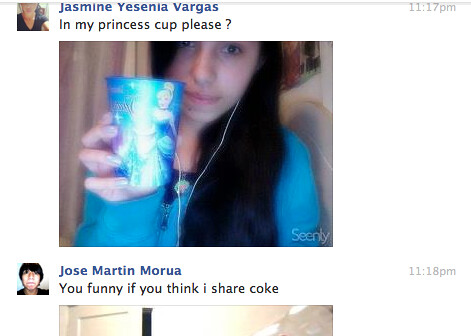The screenshot features social media posts from two users. The first post, by Jasmine Yesenia Vargas, is timestamped at 11:17 PM. Jasmine's user image shows only the bottom half of her face and chest, dressed in a black V-shaped collar shirt. Her name is written in blue, followed by the caption, "In my princess cup please?" in black text. Below her post, there's a picture of Jasmine, a woman with long black hair, wearing a blue shirt and holding a blue cup decorated with a princess pattern.

Directly below Jasmine's post is another user, Charles Martin Mara (referred to also as Jos Martin Morua in one description). His user image is a picture of a man, and his name is written in blue. His post, timestamped at 11:18 PM, reads in black text, "You funny if you think I share coke."